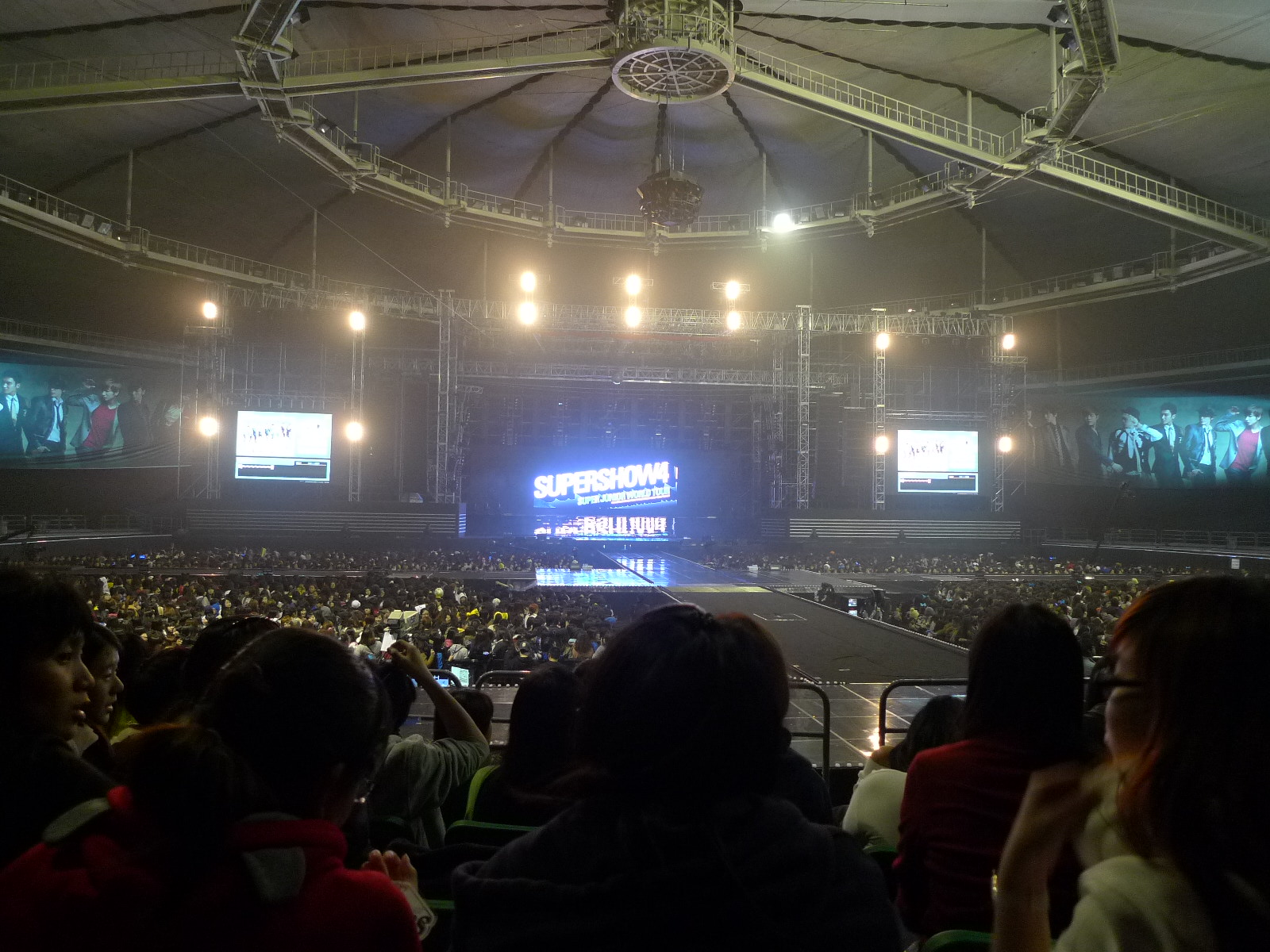A panoramic photograph captures an expansive auditorium or arena filled with an eager audience, all facing a prominent stage adorned with a blue backdrop displaying the words "Super Show 4." The venue boasts a roof with a gracefully curved, tender design that accentuates its architectural elegance. On either side of the stage, large screens display images of four young men, hinting at the performers for the upcoming event. The atmosphere is electric with anticipation, as the stage remains empty, with attendees eagerly waiting for the show to commence. Extending from the stage is a long runway that reaches out into the center of the crowd, promising an immersive and engaging performance experience.